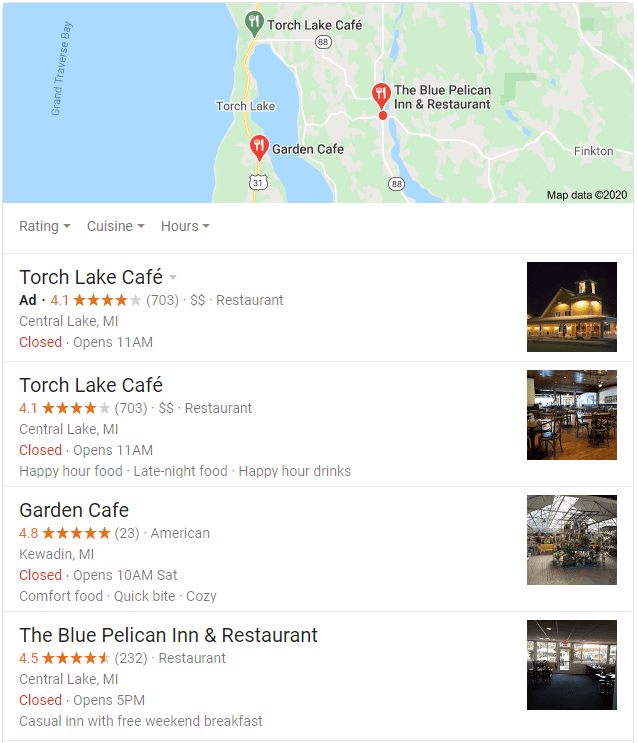The image displays a detailed map from a map website highlighting several landmarks and vacation spots in the area surrounding Torch Lake. The map provides directions to Torch Lake Cafe, Torch Lake Garden Cafe, and the Blue Pelican Inn and Restaurant, all located along Route 88 and Route 31 near the town of Finkton. The map is primarily focused on the vicinity of Torch Lake, a significant blue body of water in the region.

Below the map, there are details about Torch Lake Cafe, a four-star restaurant located in Central Lake, Michigan. The cafe is currently closed but opens at 11 a.m. It features ratings, cuisine categories like happy hour food, late night food, and happy hour drinks. There is an accompanying photograph of the cafe beside its listing.

Next, the Garden Cafe, another highly-rated eatery with a 4.8-star rating from 23 reviewers, is shown. This American restaurant is situated in Keweenan, Michigan, and is also currently closed, with plans to open at 10 a.m. on Saturday. It is known for comfort food, quick bites, and a cozy atmosphere, with a related photo also provided.

Finally, the Blue Pelican Inn and Restaurant, boasting a 4.5-star rating from 232 reviews, is located in Central Lake, Michigan. This casual inn, which offers a free weekend breakfast, is closed at the moment and will open at 5 p.m. A darker photograph of the inn is included in its directory listing.

Overall, the listings provide comprehensive information about the operating hours, star ratings, culinary offerings, and visual depictions of each establishment, catering to potential visitors planning their dining experiences in the Torch Lake area.